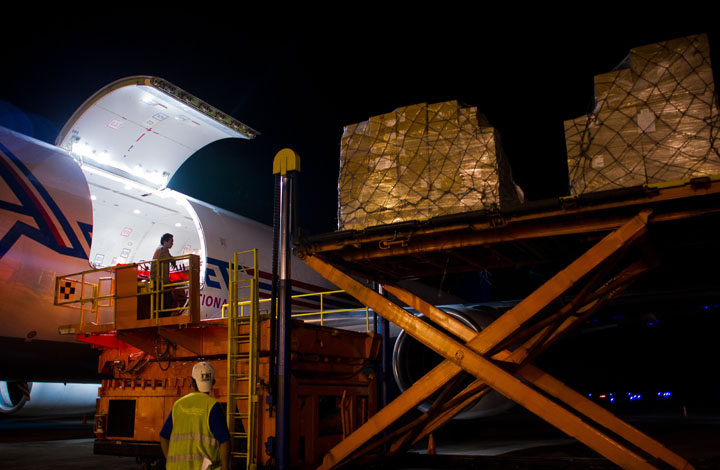The photograph captures the nighttime loading process of a white commercial cargo plane. Illuminated from within, the plane's hatchback door is open, revealing its lit interior. An orange lift with yellow rails and ladder is positioned beside the plane, supporting tightly shrink-wrapped brown cardboard boxes secured with black wire mesh. These packages rest on pallets ready to be loaded into the plane. To the bottom left, a man with a backward white cap, short dark hair, and a yellow safety vest over a blue undershirt stands with his back turned to the camera, overseeing the operation. The background fades into a dark, night sky. A partially visible logo in blue and red on the plane hints at the airline's branding, though the open hatch obscures most of it.